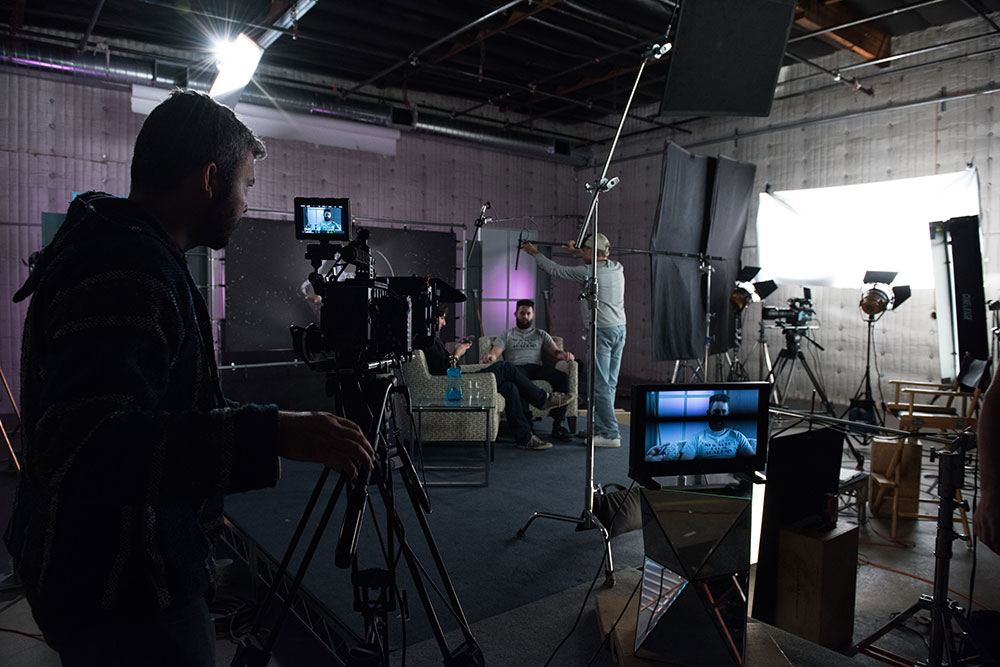This detailed photograph captures a bustling film or live action set within a large, soundproof studio featuring high ceilings adorned with exposed steel latticework for hanging lights. The walls are padded in a gray or off-white shade to enhance sound quality. The set is well-equipped with multiple cameras, tripods, various lights both floor-mounted and ceiling-hung, and numerous screens displaying live footage of the scene. 

In the foreground, a cameraman, partially shadowed, diligently captures the action on a large camera, pointing towards two living room-style chairs. One chair is occupied by a man, while the other appears to have someone partly obscured. Nearby, another crew member hoists a long-pole microphone overhead to record audio, highlighting the collaborative nature of the setup. 

Visible in the backdrop, a large white sheet is fixed to the padded wall and illuminated by spotlights, possibly serving as a backdrop or reflector. The expansive room and intricate setup, including perhaps some sort of scaffolding and additional equipment like deflector screens, signify a meticulously organized studio environment, likely staging an interview or talk show segment.